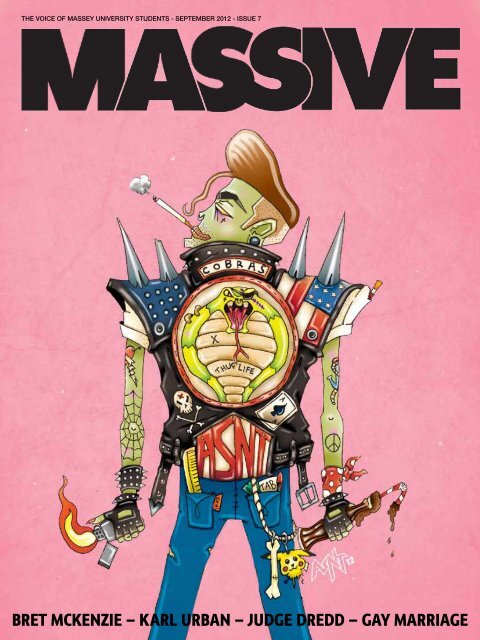The image depicts a pink promotional poster that serves as the front cover of a magazine titled "MASSIVE." At the very top, in fine print, it reads, “The Voice of Massey University Students, September 2012, Issue 7.” The word “MASSIVE” dominates the upper section of the poster in large capital letters. Below this title is an illustration of a punk-styled character with distinctive features: the character is adorned in blue denim jeans, a leather jacket with spikes on the shoulders over a white T-shirt, and tattoos covering their bare green arms and face. The character sports a rocker punk hairstyle with brown hair and sideburns, a curl draping over the face, and is depicted with their back turned, head turned towards the viewer, and smoking a cigarette.

The jacket features several adornments, notably the word “Cobras” written in small letters with an illustration of two cobras entwined beneath it, tongues extended. In the middle of the character's back are the red capital letters “A-S-N-T.” The jacket is further adorned with various memorabilia, including a small Pikachu hanging from a belt or tassel. The character's hands hold a lit Zippo lighter and a bottle of soda with a straw, respectively. Additional details include studded bracelets, gloves, and nail polish. At the bottom of the poster, names such as Brett McKenzie, Carl Urban, Judge Dredd, and references to “Gay Marriage” are listed, suggesting topics covered in this issue.